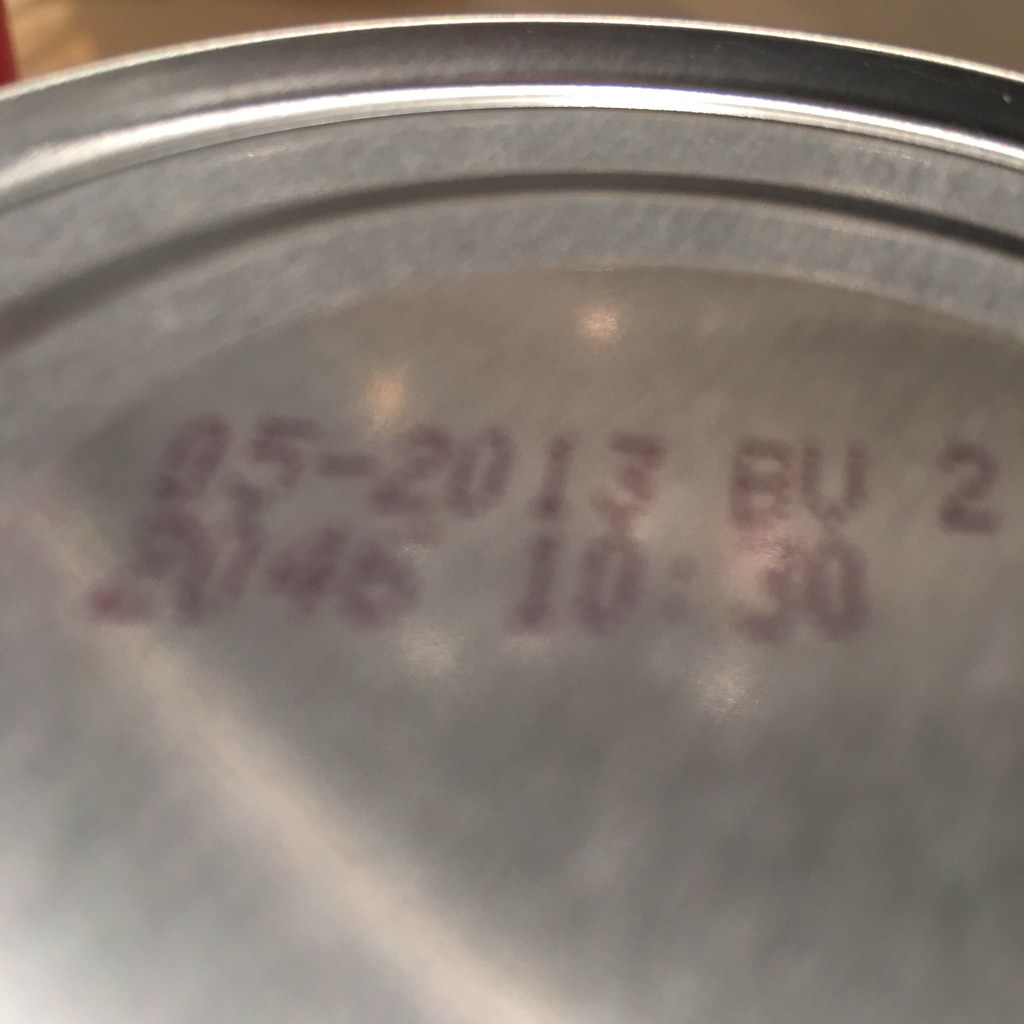This is a close-up color photograph of the top of a can, taken at an angle that focuses primarily on the lid. The image is somewhat blurry, adding a subtle abstract quality to the depiction. At the very top edge, a hint of brown color is visible, suggesting surrounding elements outside the frame. A small section of red can be seen in the left-hand corner, providing a contrasting splash of color.

The upper surface of the can is prominently featured, characterized by its silver metallic edge. Yellow reflections dance across the surface, likely from ambient light sources. A distinct line runs from the center left to the middle center of the can’s top, adorned with red text that likely indicates important information.

Clearly printed are two sets of characters: “05/2013 BU2” appears at the top, while directly below reads “204610:30.” These alphanumeric markings suggest they represent either manufacturing or expiration dates, providing key details about the product's timeline. The rest of the photograph is devoid of any other elements, ensuring that the viewer's attention is firmly held by the detailed, albeit slightly obscure, information on the can's lid.